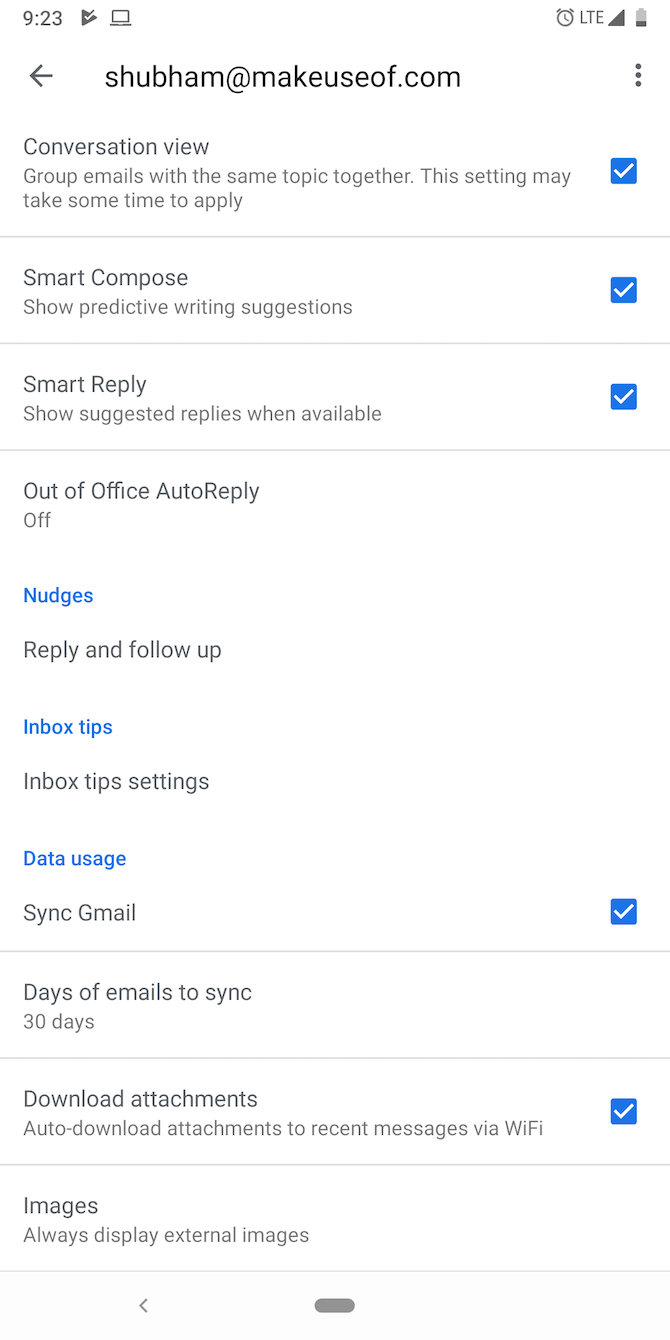The screenshot depicts a section of a website, featuring various settings and options, all set against a white background. At the top of the screen, the number "923" is displayed next to a triangle icon containing a check mark. Beside these, there's an icon of a computer or laptop. On the right side, there are icons for an alarm clock, LTE signal, cell signal strength, and battery life indicator.

Moving down, a left arrow is visible along with the text "Shubham at makeuseof.com" ("Shubham" being "SHUBHAM" and "makeuseof" written as "make use of"). To the right of this text, three vertical dots are present, likely indicating more options.

Further down, the text "Conversation View" is displayed, followed by an explanation that group emails will be grouped together based on their topic, and a note that the settings may take some time to apply. Alongside these options are blue squares with white check marks inside.

The next setting is "Smart Compose," which enables predictive writing suggestions, and below it, "Smart Reply," showing suggested replies when available. "Out of Office Auto Reply" is currently set to off.

The term "Nudges" is highlighted in blue, indicating it may be an actionable or clickable item encouraging follow-up on emails.

Next, "Inbox Tip Settings" and "Data Usage" are also in blue text, implying they are interactive options. "Sync Gmail" is displayed in regular black text. Following that, "Days of Emails to Sync" is set to 30 days. Lastly, the option "Download Attachments" and the setting to "Always Display External Images" are mentioned, indicating the user's preferences for handling attachments and images.